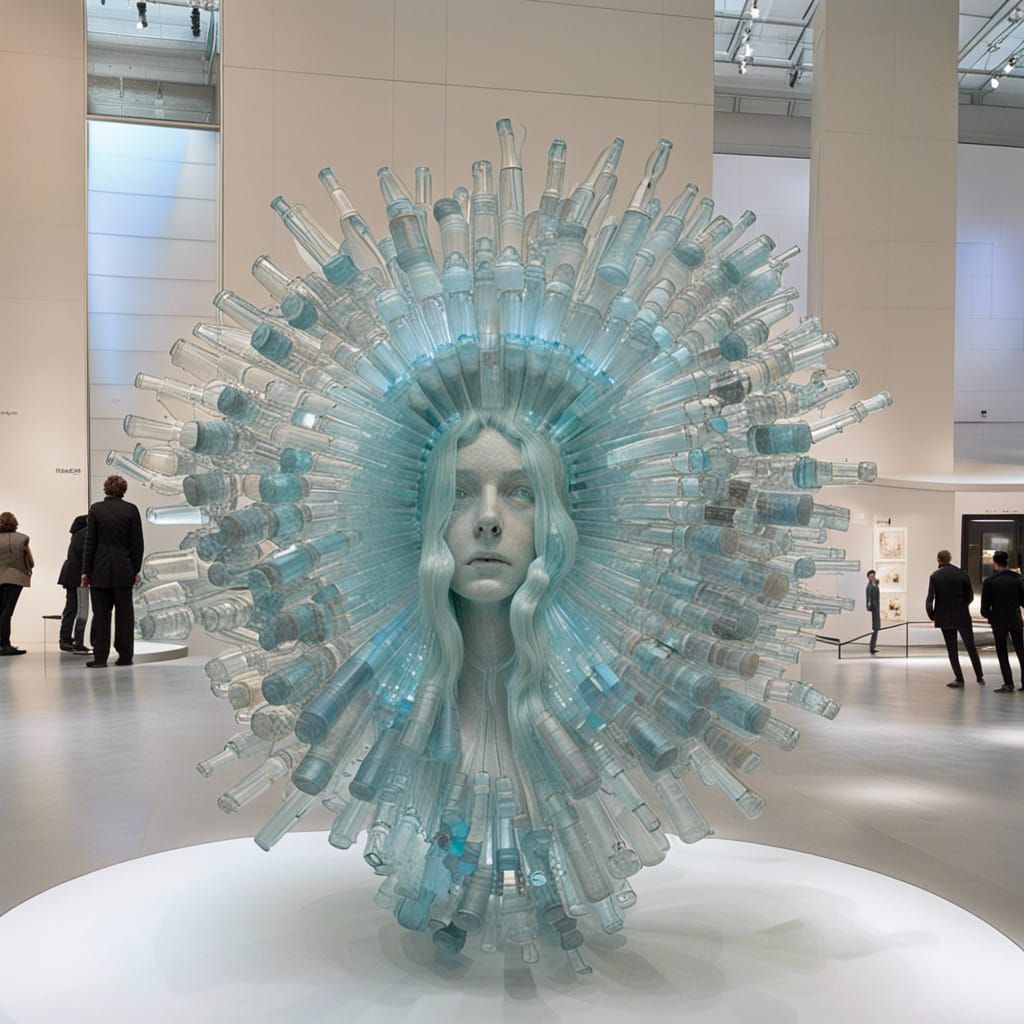This image showcases an intricate art piece displayed in an art museum with towering white walls and individuals observing various exhibits in the background. The focal point is a hyper-realistic sculpture of a woman's head with wavy, blonde hair cascading around her face. Her skin has a white, plastic-like finish, and she gazes upward with a serious expression. Surrounding her head are multiple layers of transparent glass bottles with blue labels and different sizes and shapes, some placed upside down, creating an icy, halo-like effect. The sculpture rests on a round white base. The bottles radiate outwards in all directions, enhancing the ethereal, almost otherworldly ambiance of the piece.